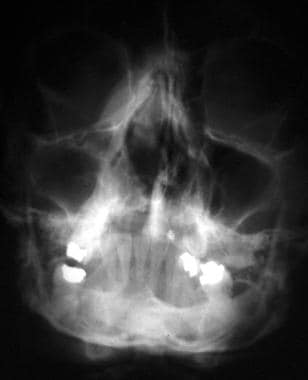The image depicts a black-and-white x-ray of the front of a person's face with a black background. The x-ray distinctly shows the nose, mouth, and jaw, with clear visibility of the teeth, including several glowing areas that might indicate capped teeth or fillings which are shining prominently. The nasal cavity and sinus areas are also visible. The overall figure inside the black background exhibits shades of white and gray, with the x-ray structure being slightly circular with a triangular shape at the top representing the nose. Additionally, two darker, possibly open, circular sections are seen on the left and right sides, contributing to the detailed anatomical view. The image has low illumination, highlighting the high contrast typical in x-ray imaging.